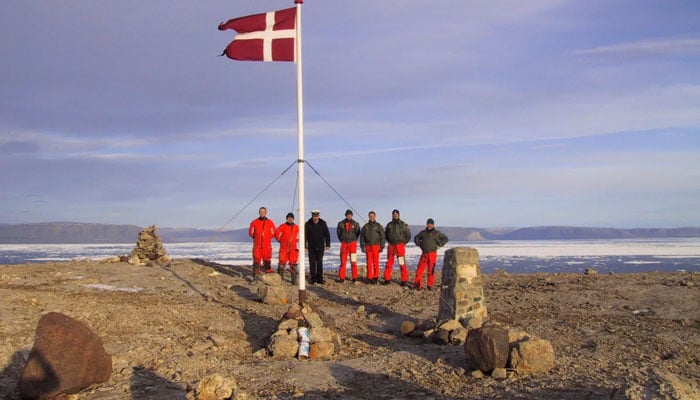The image showcases a stunning backdrop of a vivid blue sky adorned with scattered white clouds. Below, the expansive ocean stretches out, its surface punctuated by frothy white waves. In the foreground lies a rugged field, strewn with rocks, dirt, and patches of mud. Dominating this scene is a tall flagpole, proudly hoisting a red flag emblazoned with a white cross at its center.

In front of the flagpole, seven men are meticulously arranged in a line. Four of them are clad in gray jackets paired with orange pants, creating a striking contrast with their surroundings. At the center of the lineup stands a man dressed entirely in a black uniform, complemented by a white naval-style cap. Flanking this central figure are two gentlemen donning long orange coats, adding a splash of vibrant color to the assembly. This tableau captures a moment of striking visual and thematic contrast.